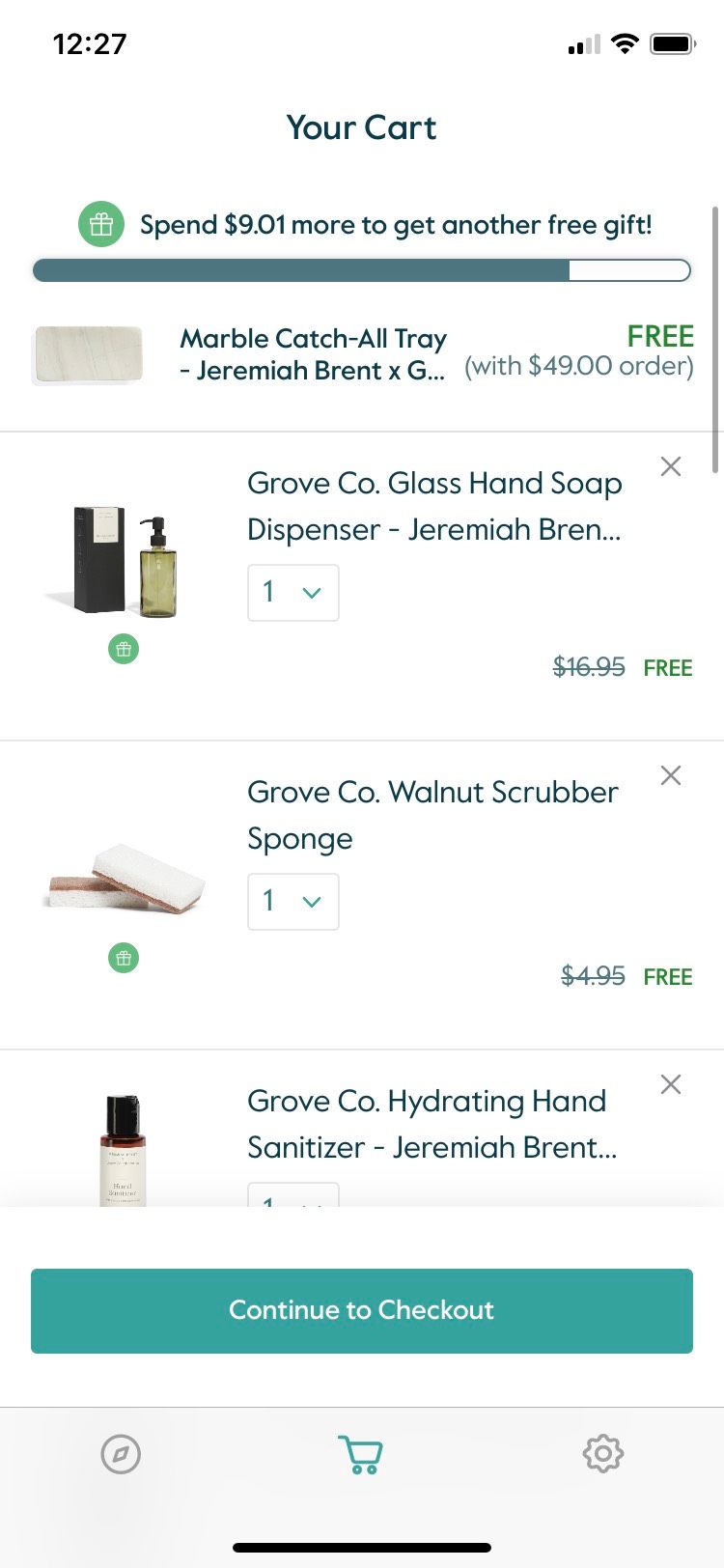A detailed screenshot of a shopping app displayed on a smartphone. The top of the screen shows a time of 12:27, with a WiFi symbol indicating full connectivity and a fully charged battery icon. Below it, the shopping cart icon is present with a green circle; marked "92" indicating 92 items. The brand displayed is "Jeremiah Brand," and the cart is mostly full. A message states "Free with a $49 order," and an option to add more items to receive a free gift. 

A specific item, "Marble Catch-All Tray," appears multiple times. Other items include a "Grove Company Glass," and another Jeremiah Brand product, a black pump bottle. There's a notation for a $16.95 price, crossed out, indicating a discount.

A blue rectangle with white text in the center, possibly an ad or special offer, is visible. Navigation elements include a compass icon for location-based offers at the bottom, a cart icon, a gear icon on the bottom right for settings, and a sign-in option at the bottom. The right-hand side shows a scroll bar, currently at the top. The interface is in light theme mode, and the screen's pull-up line at the bottom indicates it is in portrait orientation.